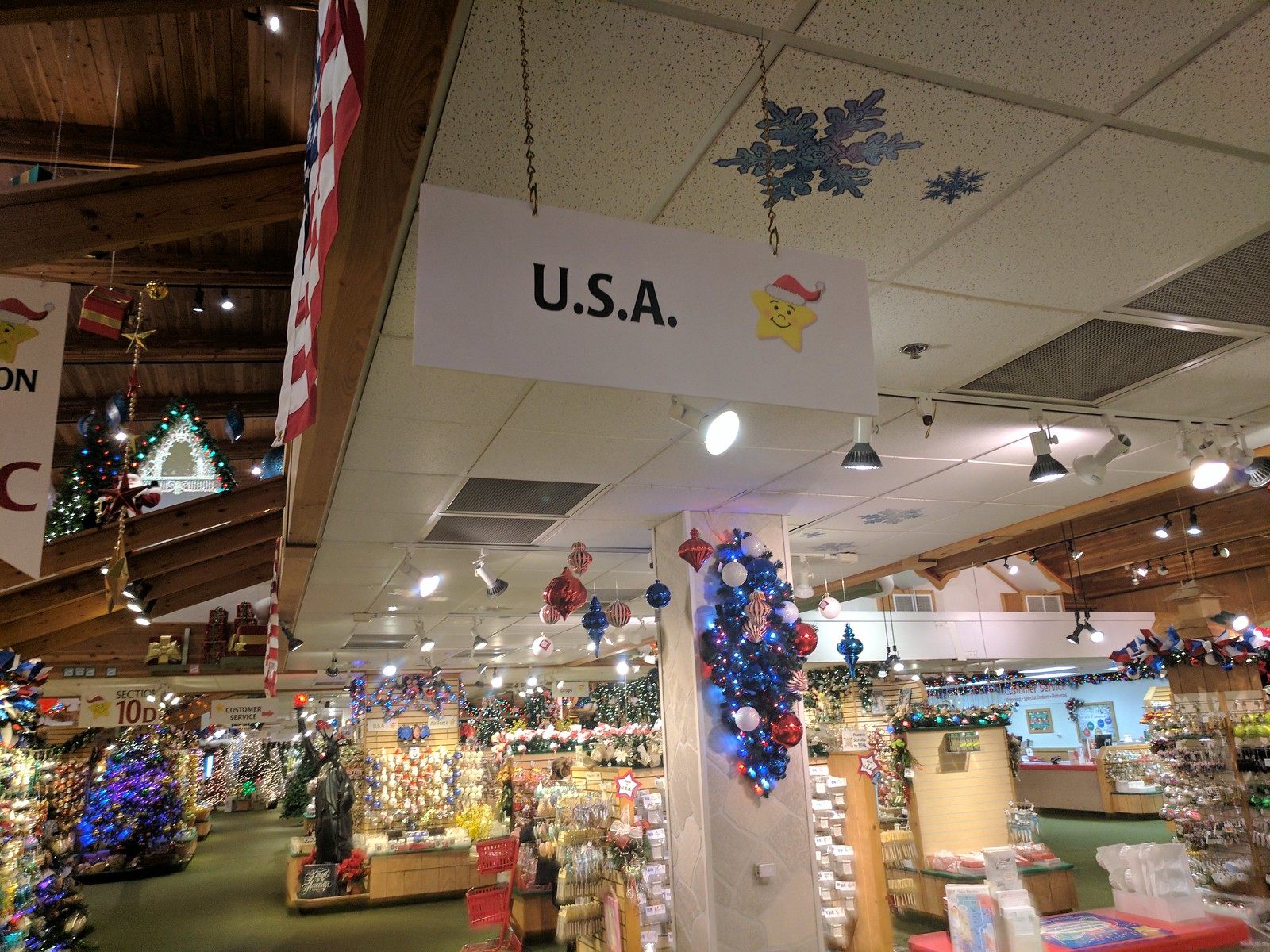An expansive store, potentially a department store like Macy's, is adorned with festive Christmas decorations. On the left, a brilliantly lit Christmas tree with blue lights stands out against the holiday-themed backdrop. Suspended from the ceiling is a sign that reads "USA," featuring a star embellished with a Santa hat, further accentuating the Christmas atmosphere. The store is filled with various stands displaying items for sale, reminiscent of a bustling gift shop. Towards the back, a customer service desk is visible, illuminated by numerous hanging lights, contributing to the overall festive ambiance.